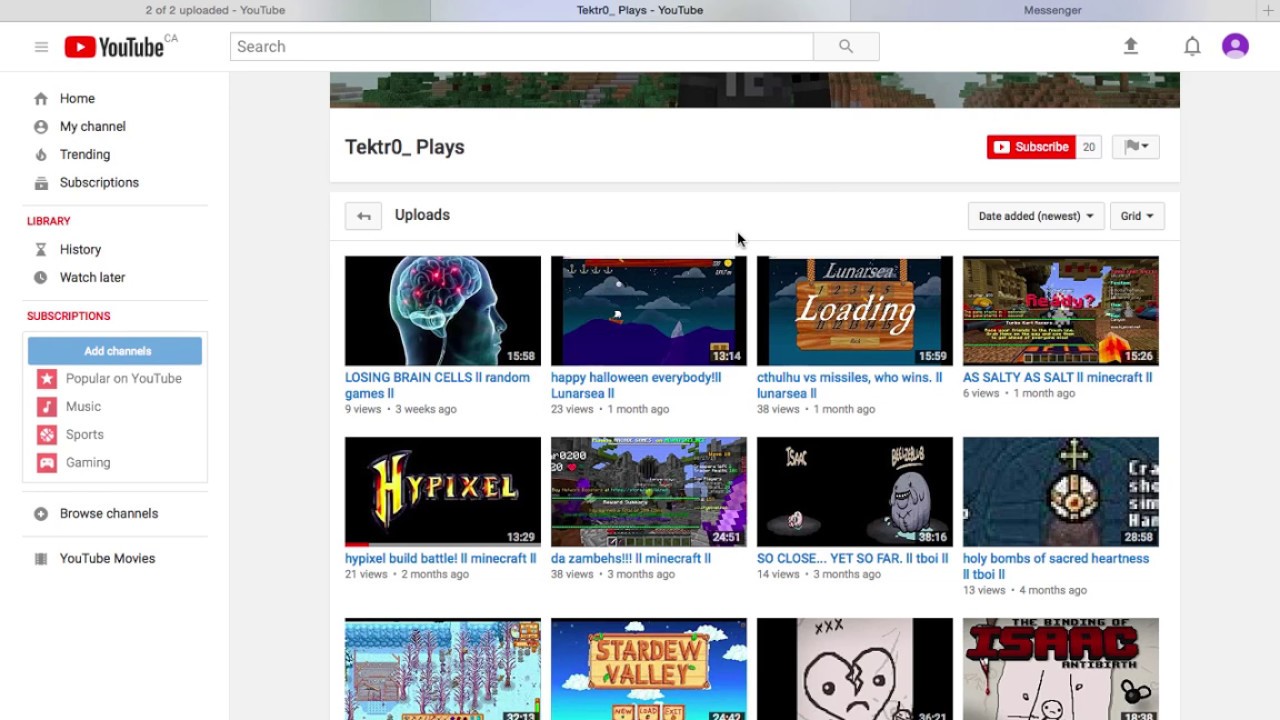The image shows a detailed screenshot of a YouTube interface with multiple tabs and sections open. The browser border at the top is gray, indicating three open tabs. The first tab, labeled "2 of 2 uploaded - YouTube," is dark gray. A second tab in black reads "TEKTR0_plays - YouTube," and the third one is labeled "Messenger."

Below the tabs, the left sidebar features a white background. At the very top of this sidebar, there's a small gray label with the letters "CA" followed by the prominent YouTube logo in black next to three horizontal gray lines. 

Underneath a thin gray line that stretches horizontally, there are several navigation options in black: "Home," "My Channel," "Trending," and "Subscriptions." Another thin gray line follows, leading to a section labeled in red: "Library." Below "Library," the options "History" and "Watch Later" are listed in black.

Another thin gray line divides sections, after which "Subscriptions" is highlighted in red with a corresponding square box next to it. Within this box, the top portion is blue, containing the white text "Add channels" below which the title "Popular on YouTube" appears. This section further categorizes popular content into "Music," "Sport," and "Gaming" in black text, alongside a circular icon with a white plus sign.

The sidebar ends with labels "Browse Channels" and "YouTube Movies" in black. At the very top of the image, there is a white rectangle with a gray border representing a search box that has the placeholder "Search" in gray.

The main content area displays several video titles and their respective details in white text: "Losing Brain Cells - Random Games" (15 minutes, 58 seconds), "Happy Halloween, Everybody - LunarC" (13 minutes, 14 seconds), and "So Close Yet So Far" (38 minutes, 16 seconds).